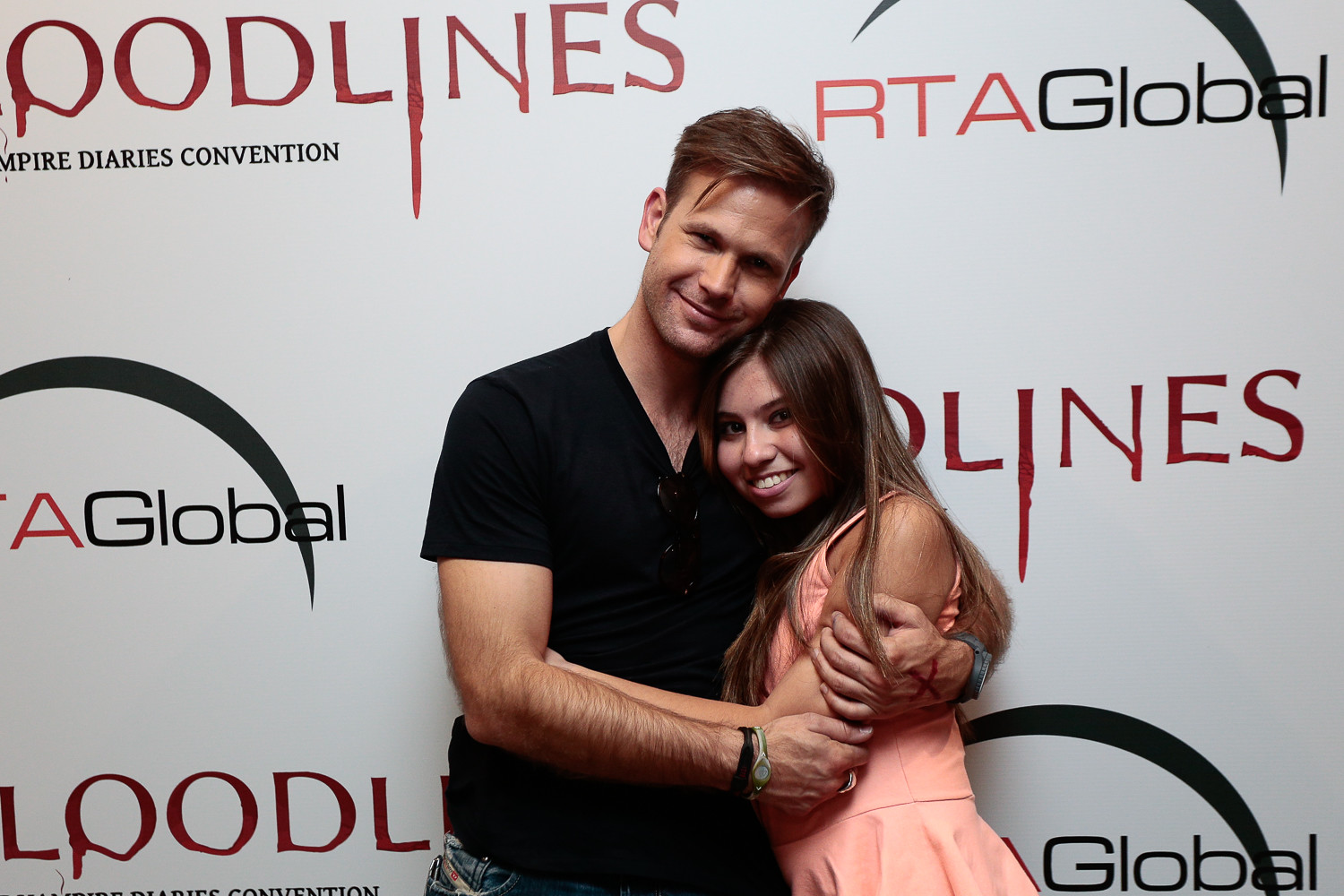In the center of the image, a man and woman embrace warmly, smiling directly at the camera. The man, with brown hair, wears a black v-neck t-shirt and blue jeans. His wrists are adorned with several items, including a watch on his left wrist, and sunglasses hang from his shirt collar. The woman, with long brown hair reaching almost to her elbows, is dressed in a pink, sleeveless dress or skirt. Both are hugging each other closely, with the man's arm wrapped around the woman's back. Behind them is a predominantly white backdrop with repeating text that reads "RTA Global" in red and black, and "Bloodlines Vampire Diaries Convention" in dark red and black, adding a thematic touch with the word 'Bloodlines' featuring a dripping blood effect.